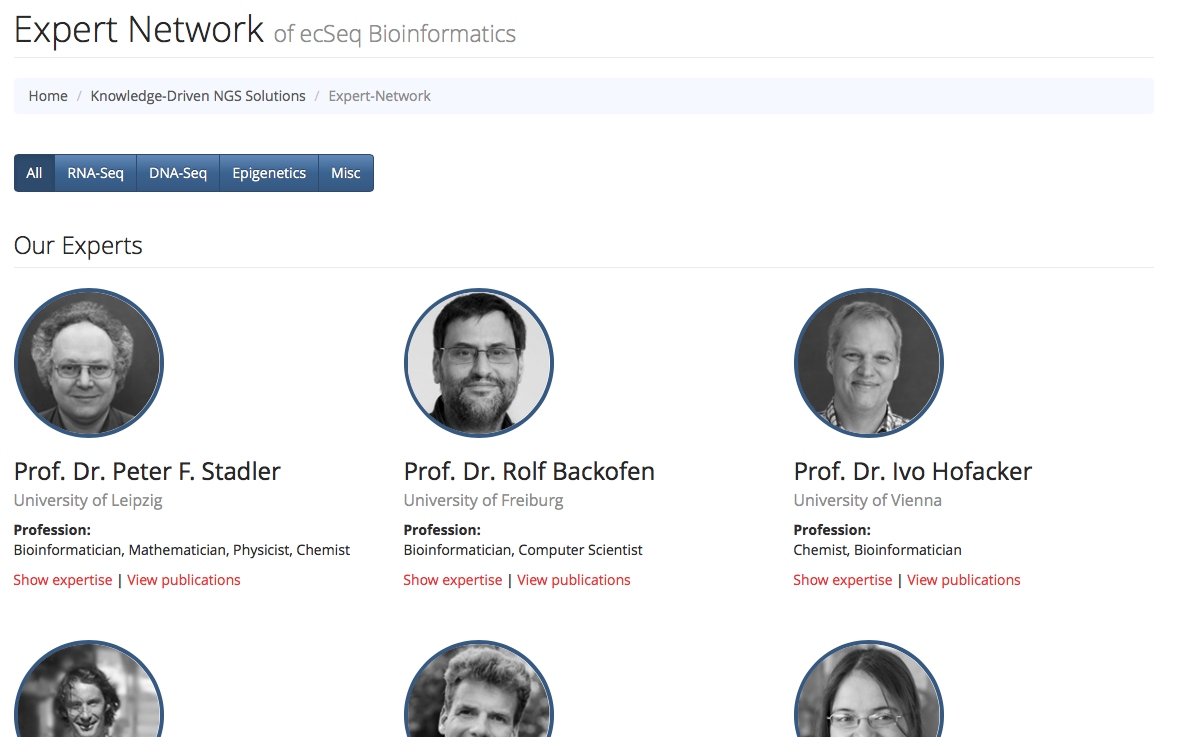This screen capture features a section of a webpage dedicated to highlighting profiles of distinguished professors involved in bioinformatics. The webpage, set against a clean white background, belongs to the "Expert Network of EC-SEQ Bioinformatics." 

At the top, visible text includes a file path: Home > Knowledge Driven NGS Solutions > Expert Network. Below this, a blue menu bar with white text offers clickable categories: All, RNA Sequence, DNA Sequence, Epigenetics, and Miscellaneous. 

The section is titled "Our Experts" and is followed by six headshots. Each headshot is presented in a blue-outlined circle with black and white photographs of the professors. 

In the top row of three:
1. Professor Dr. Peter F. Stadler from the University of Leipzig. His professions are listed as Bioinformatician, Mathematician, Physicist, and Chemist. The text provides further options to "Show Expertise" and "View Publications."
2. Professor Dr. Rolf Beckhofen from the University of Freiburg. His professions include Bioinformatician and Computer Scientist.
3. Professor Dr. Ivo Hofacker from the University of Vienna, whose professions are listed as Chemist and Bioinformatician.

The bottom row of three headshots is partially visible but cut off, preventing any textual details from being read clearly.